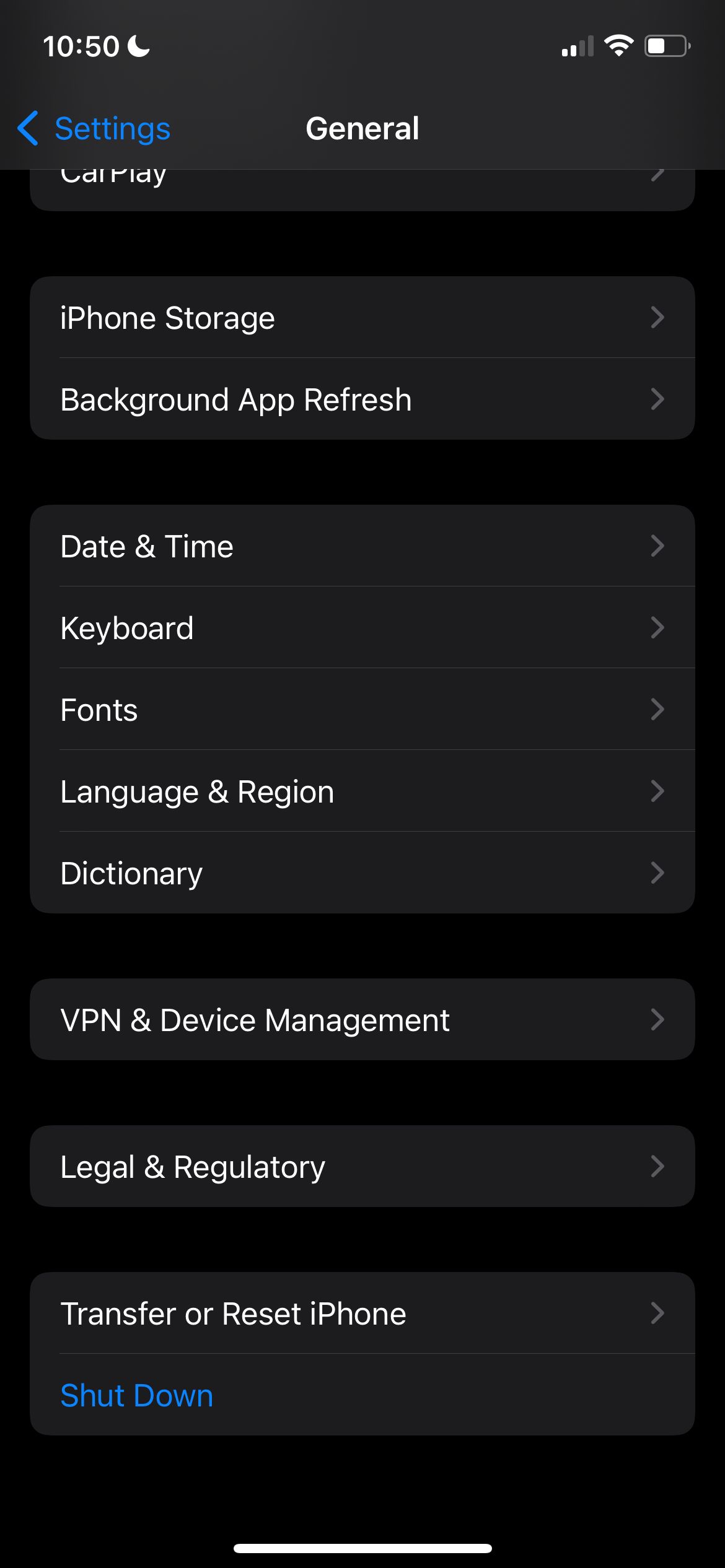This detailed screenshot captures an iPhone settings screen. At the top, the time displayed is 10:50, accompanied by a moon icon indicating the "Do Not Disturb" mode is active. The battery icon shows roughly 50% charge remaining. The network indicators at the top right reveal a fully shaded Wi-Fi signal and a cellular signal with two out of four bars.

The screen displays the "Settings" menu with a black background, featuring several options in blue text. These include:

- iPhone Storage
- Background App Refresh
- Date & Time
- Keyboard
- Fonts
- Language & Region
- Dictionary
- VPN (with "V," "P," and "N" capitalized)
- Device Management
- Legal & Regulatory
- Transfer or Reset iPhone, with "Shut Down" listed underneath this heading.

At the bottom middle of the screen, a white bar is visible, indicative of the navigation slider.